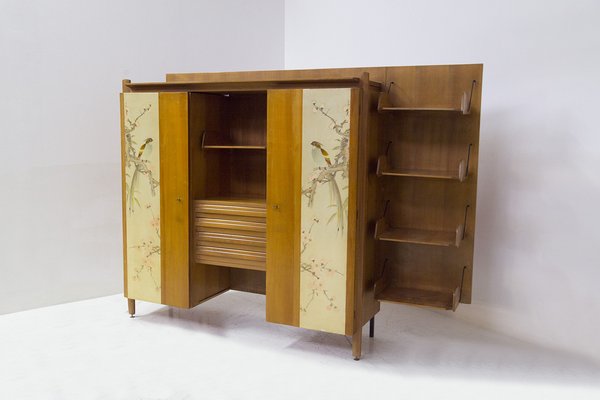A beautifully designed wooden cabinet, adorned with an Eastern-inspired aesthetic, stands prominently in the corner of a pristine white room. The cabinet features intricate scroll designs that exhibit a delicate beige color, enhanced with detailed illustrations of plants and birds. Centered on the cabinet's doors are captivating images of birds with long tails and brown backs, perched thoughtfully on branches. These illustrations are meticulously painted on scrolls that draw attention toward the middle of the cabinet. The doors of the cabinet are slightly ajar, revealing the inner structure which comprises a single shelf at the top, and below it, several shelves or drawers, hinting at ample storage space. To the right side of the cabinet, additional shelving is attached, forming part of a larger wooden wall segment that integrates seamlessly with the main structure. The cabinet casts a gentle shadow on the ground and wall, adding depth and character to the corner of the room where it resides.